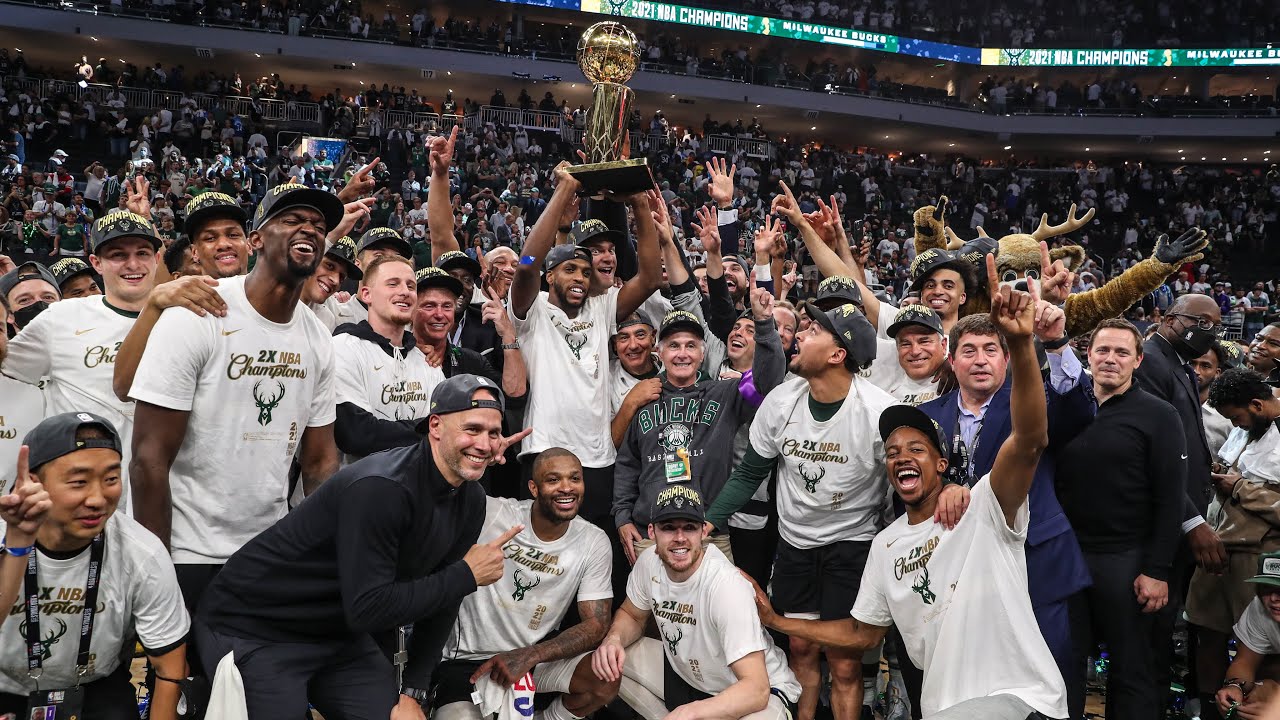In this vibrant indoor photograph taken in a basketball stadium, the jubilant Milwaukee Bucks celebrate their 2021 NBA Championship victory. Central to the image is an African American player in a white shirt, holding the gold championship trophy aloft, his cap worn backwards. Surrounding him are dozens of teammates, all wearing white T-shirts emblazoned with "2x NBA Champions" and featuring the Bucks’ iconic deer logo. The coach, an older man in a gray Bucks hoodie, stands prominently among them. In the background, the Bucks' mascot, easily identifiable by his large head and antlers, raises his arms in celebration. Rows of ecstatic fans fill the stands, with a digital banner above them displaying "2021 NBA Champions, Milwaukee Bucks."